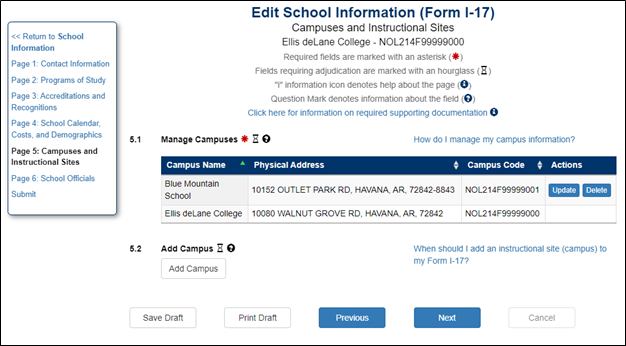**Return to School Information Form Overview**

The image features a predominantly white background with a mixture of blue and black text, presented in an organized, structured format. On the left side of the image, a small white box with blue text reads "Return to School Information" and includes several arrows pointing to different sections: 

- Page 1: Contact Information 
- Page 2: Programs to Study
- Page 3: Accreditations and Recognitions 
- Page 4: School Calendar, Cost, and Demographics 
- Page 5: Campuses and Instructional Sites (in black)
- Page 6: School Officials 
- Followed by a submit button.

Toward the center, a larger white square with a black border is prominently displayed. In navy blue text, it states "Edit School Information (Form I-17)." Below this header, the section is labeled as "Campuses and Instructional Sites," featuring "Ellis D. Lane College" along with a unique alphanumeric campus code. 

Key instructions and icons are included for user guidance:
- Required fields are marked with a red asterisk (*).
- Fields needing adjudication are marked with an hourglass icon.
- An information icon, represented as a white “i” within a navy circle, provides help about the page.
- A question mark icon, depicted as a white question mark in a navy circle, indicates information about specific fields. 
- A blue text link reads "Click here for information on required supporting documentation."

Further instructions include:
- "Manage Campuses" tagged with a red asterisk, hourglass, and question mark icons.
- The prompt "How do I manage my campus information?"

Details of campuses mentioned in the form:
1. **Blue Mountain School**:
   - Physical Address: 10152 Outlet Park Road, Havana, Arkansas 72842-8843
   - Campus Code: (Alphanumeric)
   - Actions: [Update] [Delete] (in blue and white boxes)

2. **Ellis D. Lane College**:
   - Physical Address: 180 Walnut Grove Road, Havana, Arkansas 72842
   - Campus Code: (Alphanumeric)

Additionally, there is an option to "Add Campus" accompanied by the hourglass and question mark icons, with further guidance in blue text on when to add an instructional site to Form I-17.

At the bottom of the image, several action buttons are organized in white and gray or white and blue boxes:
- Save Draft
- Print Draft
- Previous
- Next
- Cancel